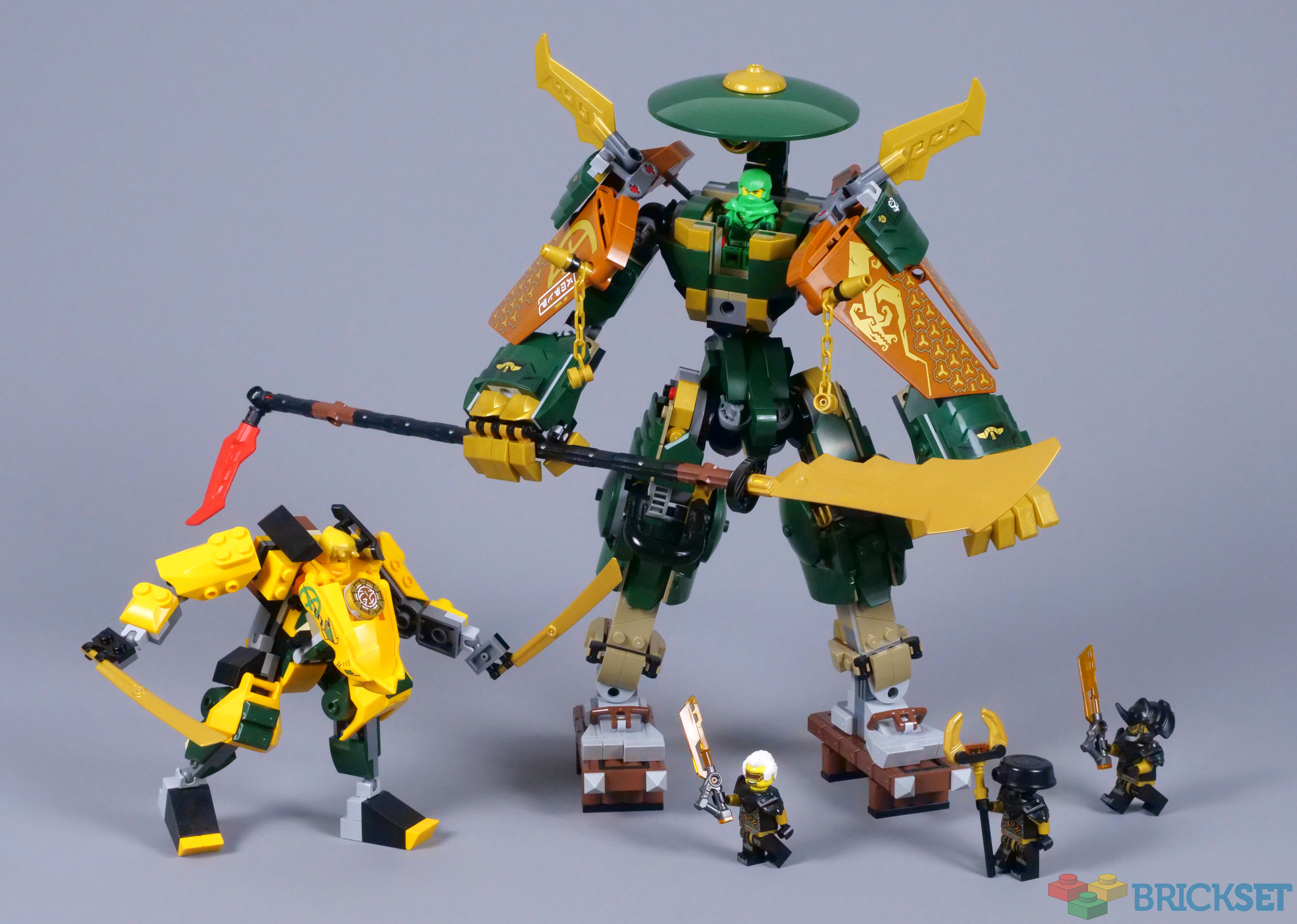The photograph displays a collection of Lego-like toys, referred to as a "Brick Set," featuring a variety of figures and constructs. At the center are two large composite figures, reminiscent of transformer creatures. The more prominent, green figure is detailed with green and orange blocks and features a flying saucer-like cockpit controlled by a small green octopus-like character. This figure wields an elaborate spear-like weapon with a yellow cutting edge, black handle, and a red flag.

Next to it stands a medium-sized yellow creature adorned with some green and black blocks, sporting a large yellow snout and wielding two knives. On the ground below, there are three smaller Lego figures dressed in black uniforms. Two wear black helmets, while the third has a white helmet. Each of these mini-figures carries a weapon, although it's unclear who are the good guys and who are the bad guys. The entire scene is set against a gray background, and the bottom right corner of the image features the "Brick Set" text and a logo with red, yellow, and green blocks.